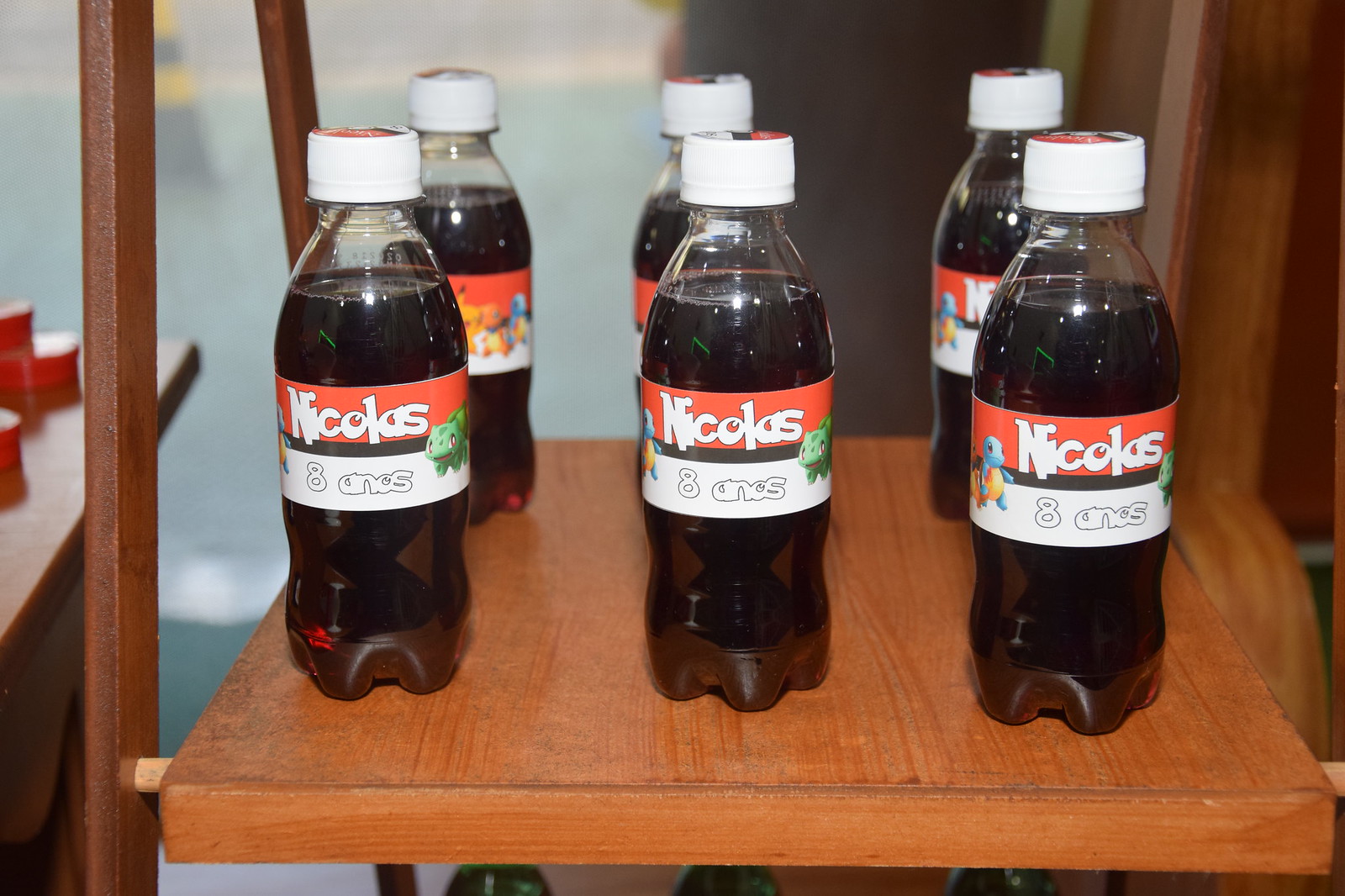The image features six clear plastic bottles of soda, labeled "Nicolas" with the number "8 Anios," positioned in two rows of three on a medium brown wooden shelf that has a triangular step design. Each bottle is filled with a dark reddish liquid and capped with a white bottle top, featuring red and blue details. The labels on the bottles are predominantly red with white lettering outlined in black, and there are illustrations of Pokémon characters—Squirtle, Bulbasaur, Charmander, and Pikachu—indicating a special collaboration or themed edition. The bottles have a celebratory appearance, possibly designed for an 8th birthday event. Surrounding the shelf, the background includes a blue floor, an out-of-focus window revealing yellow stripes like a roadway, and a table with a red unidentified object to the right.